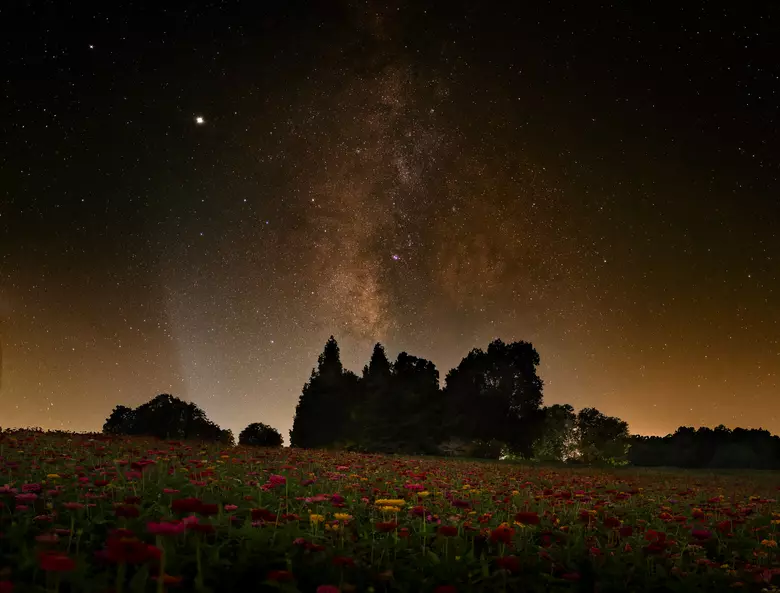The image showcases a stunning night scene set in a vibrant flowery field. In the immediate foreground, an abundance of predominantly pink flowers is interspersed with red and occasional yellow blooms. As the field extends into the background, the flowers give way to a row of trees, creating a dark silhouette against a striking orange glow. This glow suggests the remnants of a sunset, though the sun itself is not visible. Rising above the treeline, the sky transitions from a warm orange hue to a deep, bluish-black overhead. The night sky is dotted with numerous stars, including one particularly bright star in the top left and a significant pinkish-purple star within a larger cluster at the center. The right side of the sky is mostly black with a few scattered stars, contributing to the celestial ambiance of the scene. Overall, the image beautifully captures the juxtaposition of the colorful, flower-filled field and the expansive, starry night sky.